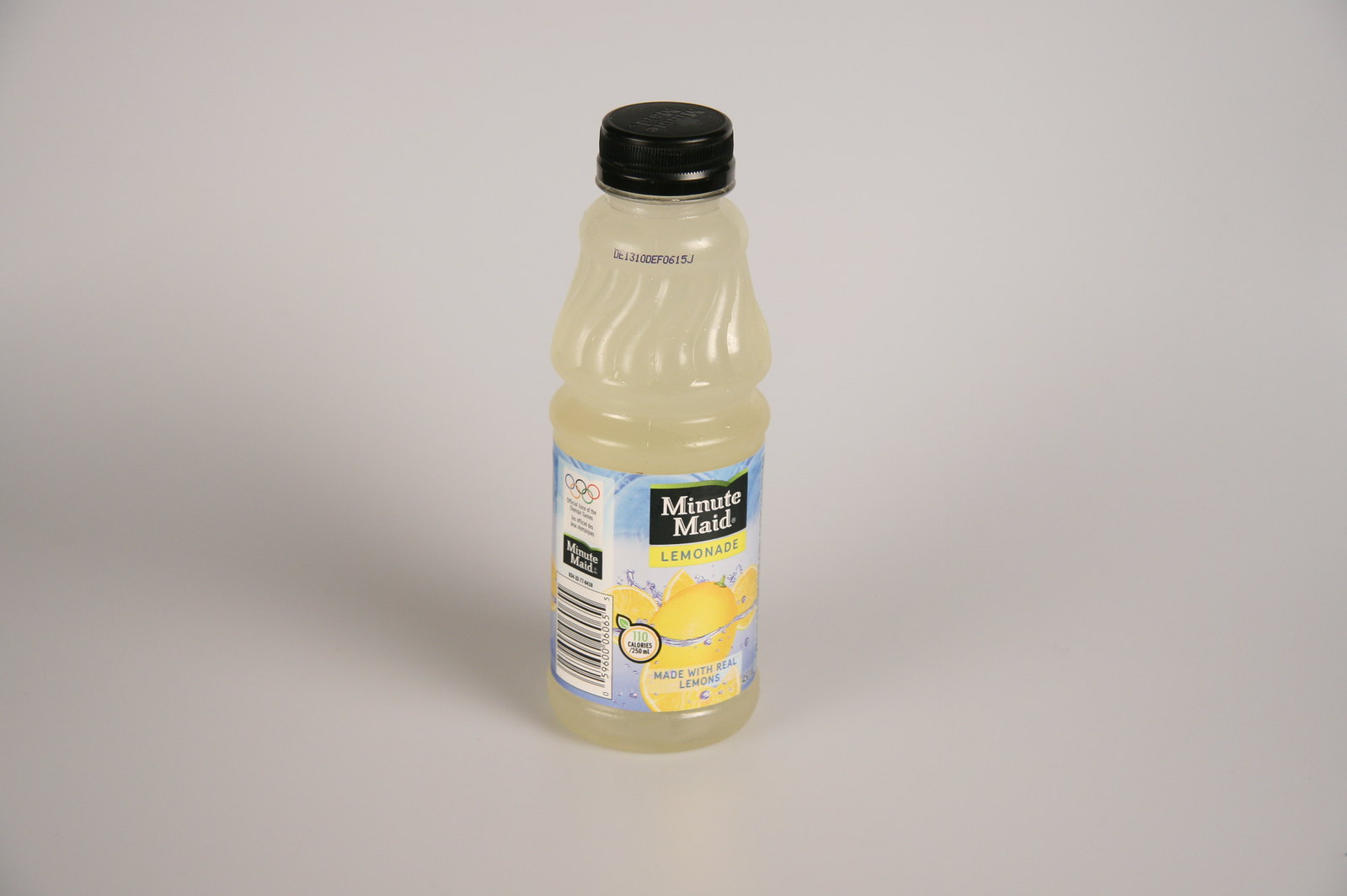The image is a color photograph of a sealed, single-serving Minute Maid lemonade bottle. The landscape-oriented image is about 30-50% wider than it is tall, and the grayish background possibly represents the surface on which the bottle sits. The lighting comes from the lower right, casting shadows to the left. The bottle is centered and stands out sharply against the white background. It features a black, screw-on cap and contains a cloudy yellow lemonade. The label, predominantly light blue with lemons depicted beneath the logos, wraps around the bottle's lower portion. The front displays the iconic Minute Maid logo in white letters on a black background, with "lemonade" written beneath it. Additional information, including a barcode and Olympic rings, appears on the side, suggesting the product's promotional tie to the Olympics. The bottle appears full, with a visible production or expiration date near the top.